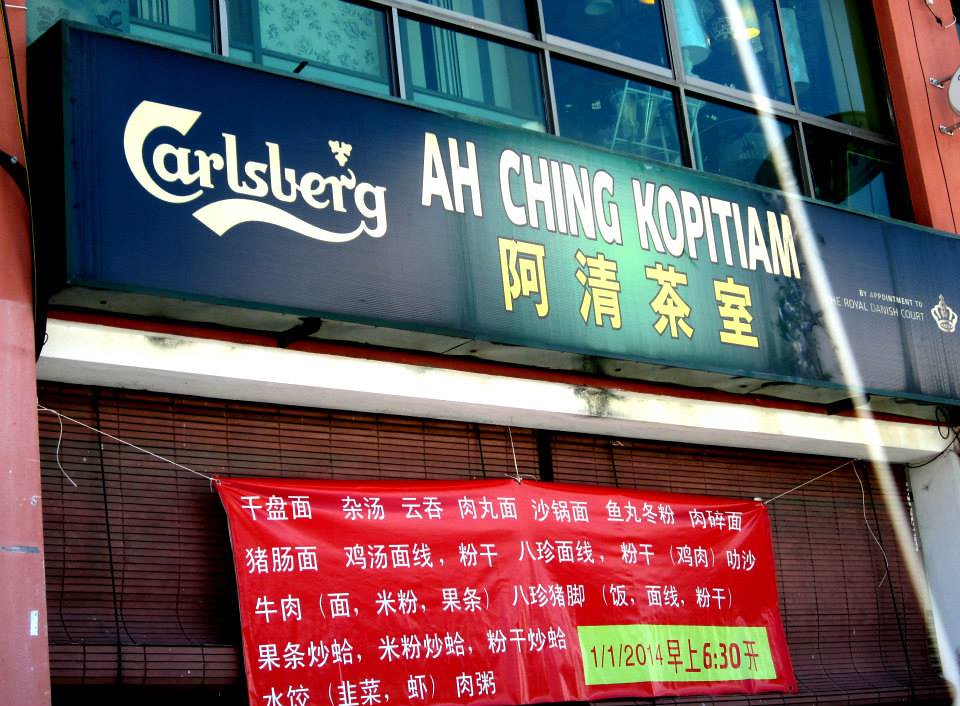The photograph captures an angled, bottom-up view of an office building that doubles as an oriental restaurant, likely named "Ah Ching Kopitiam." The focal point is a large, horizontally-aligned blue sign prominently displaying "Carlsberg" on the left, followed by “Ah Ching Kopitiam” in broad white letters, and yellow Chinese characters. Above the sign are glass windows with silver frames, showing partial reflections and a glimpse into what appears to be a residential area, possibly indicating this building serves multiple purposes. 

Below the blue sign, a red banner with white Chinese writing hangs over a bamboo curtain that closes off the restaurant’s entrance. The banner includes a combination of Chinese characters and Arabic numerals, potentially indicating a date, such as "1-1-2014" and "6-30." The bamboo curtain, dark brown in color, likely serves as the restaurant's closed doorway. Together, these elements create a vibrant and culturally rich depiction of the building's façade.